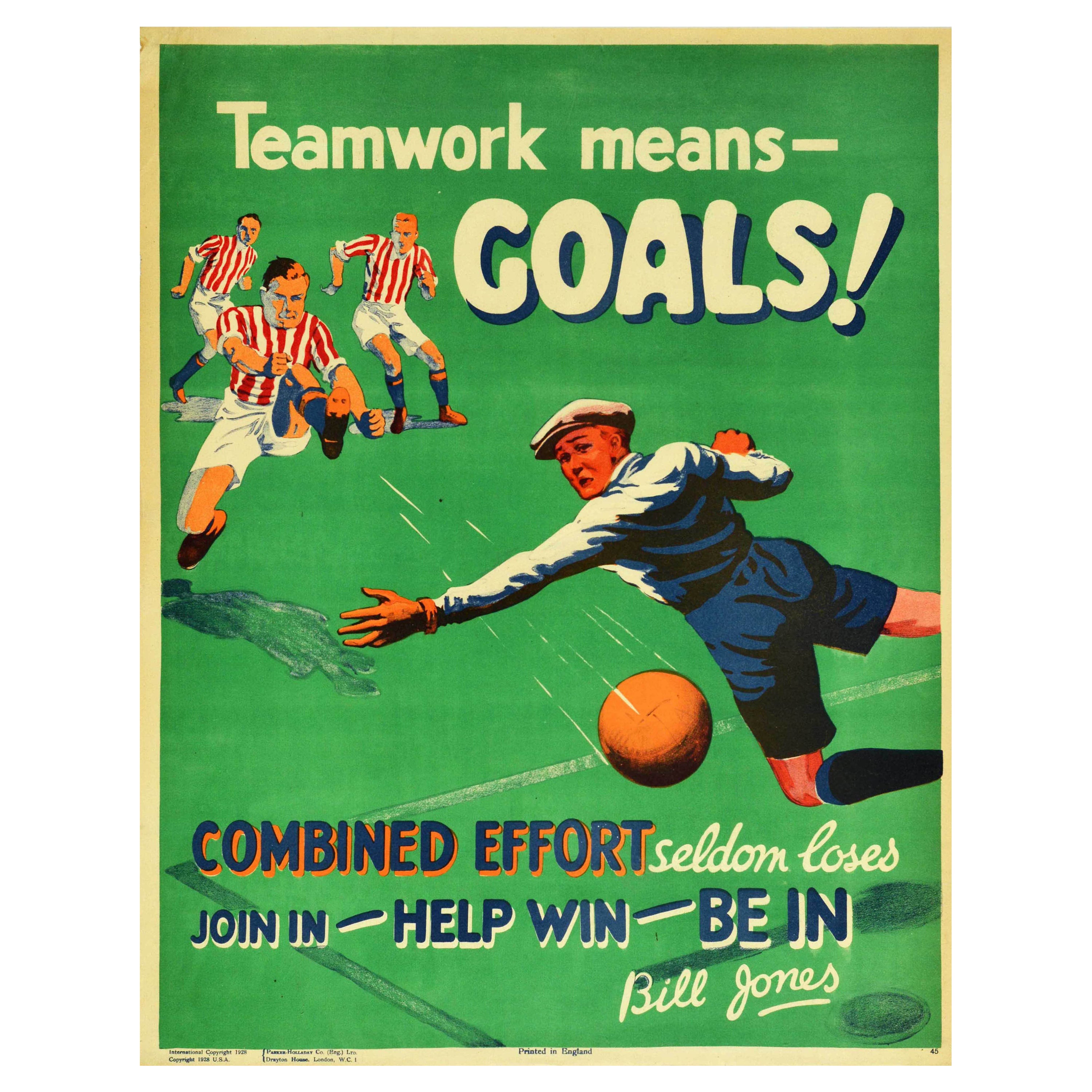This vintage poster, primarily green with a faded yellow-beige border, captures an intense soccer moment and promotes the value of teamwork. Centered at the top, bold white text with a navy blue drop shadow exclaims, "Teamwork means goals!" Three soccer players, donning red and white striped shirts and white shorts, are positioned on the left side. One player's leg is raised high, having just kicked an orange soccer ball, now hurtling towards the goal with white streaks trailing behind it. In the foreground, a goalie clad in a white upper garment, navy blue shorts, and dark blue knee pads, along with a white beret, is diving in a desperate attempt to save the ball, which he ultimately misses. To the lower right of the poster, the ball continues its path towards the goal. The bottom of the poster features encouraging text in blue and white: "Combined effort seldom loses. Join in, help win, be in." The poster is signed on the right corner in cursive by Bill Jones.